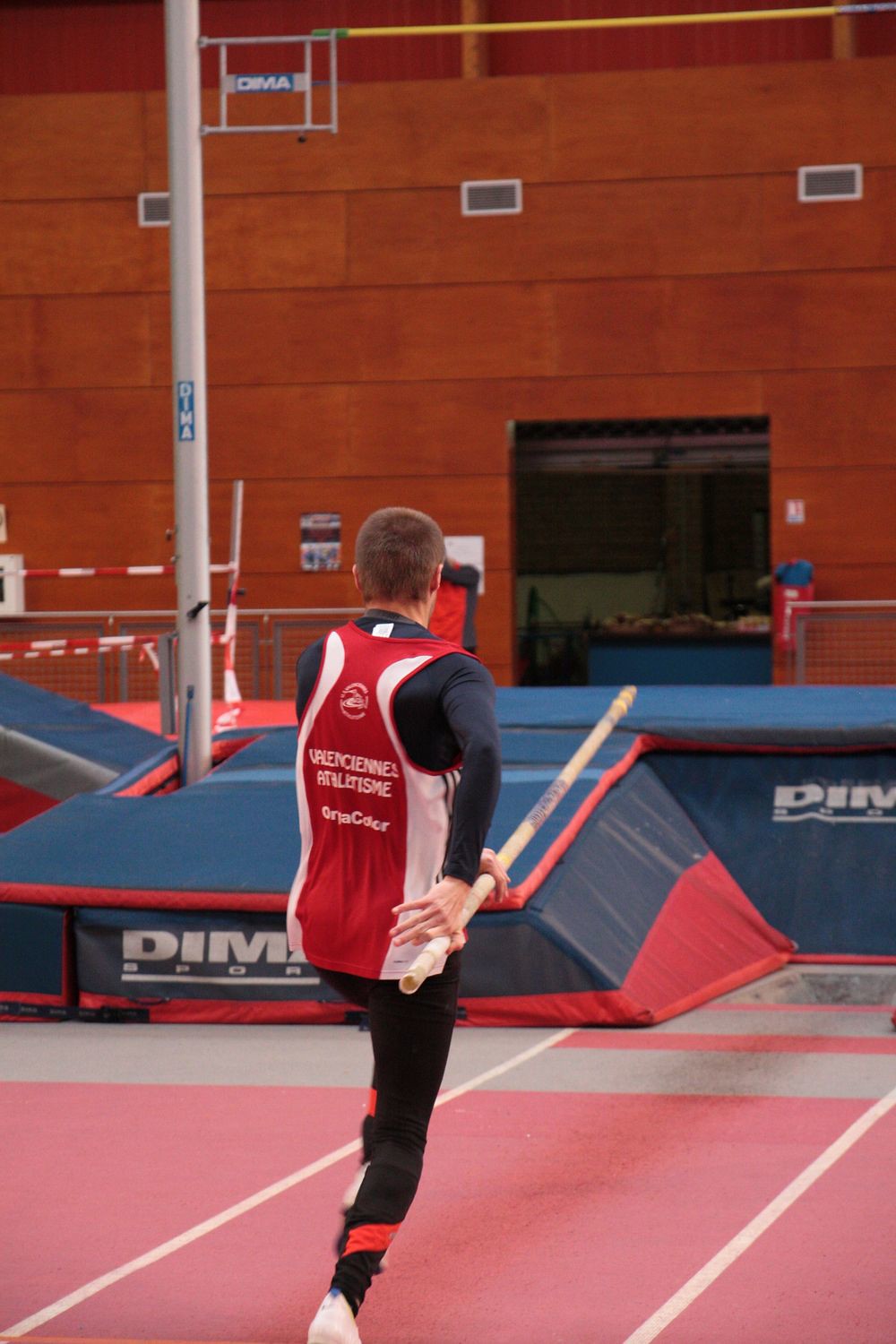In this photograph, a male athlete is captured mid-motion as he prepares for a pole vault event inside an indoor stadium. The athlete is centered in the image, wearing a distinctive red and white sleeveless jersey over a black long-sleeved shirt, emblazoned with the logo and titles "Valenciennes Athletisme." He sports black trousers with a red stripe, and white shoes. His left hand firmly grips a brown pole vault, poised for action, while his right arm is slightly behind him, indicating his imminent sprint towards the vaulting platform.

The gymnasium floor is a vivid red, marked with white lines, creating a contrast against the dark blue mats with red borders laid out beneath the vaulting area, which bear the name "DIM Sports." A horizontal yellow bar is elevated in preparation for the athlete's jump, supported by silver poles labeled "DIMA." In the background, the large red wall of the stadium features a doorway leading to an adjacent room, and the area is illuminated by several lights installed on the wall.